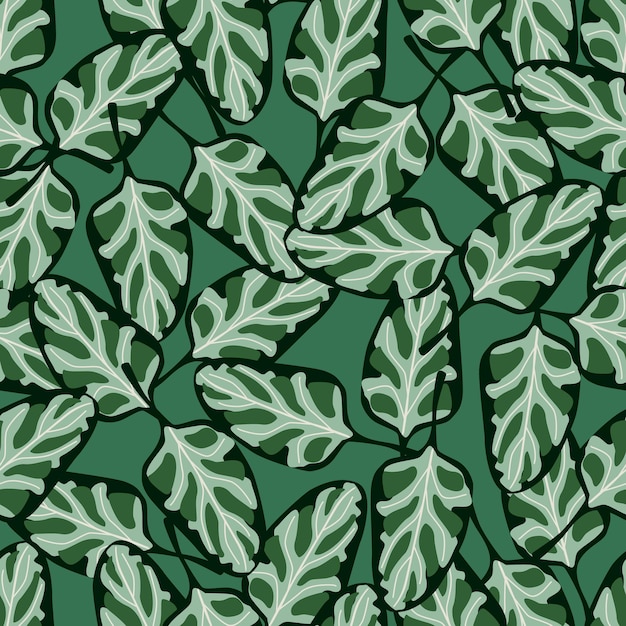The image showcases a detailed, computer-generated pattern of leaves on a forest green background. Each leaf is intricately designed with dark black or green outlines and stems, featuring a striking contrast with dark and light green hues. The veining on the leaves is prominent, with white veins branching out and surrounded by lighter green, creating a captivating contrast against the dark green areas of the leaf. The leaves are arranged in a seemingly random, non-uniform pattern, with some overlapping stems and partial views, giving a sense of depth and continuous flow across the background. The overall composition appears as a sophisticated graphic illustration, potentially suitable as wallpaper or for various design applications. There is no text within the image.